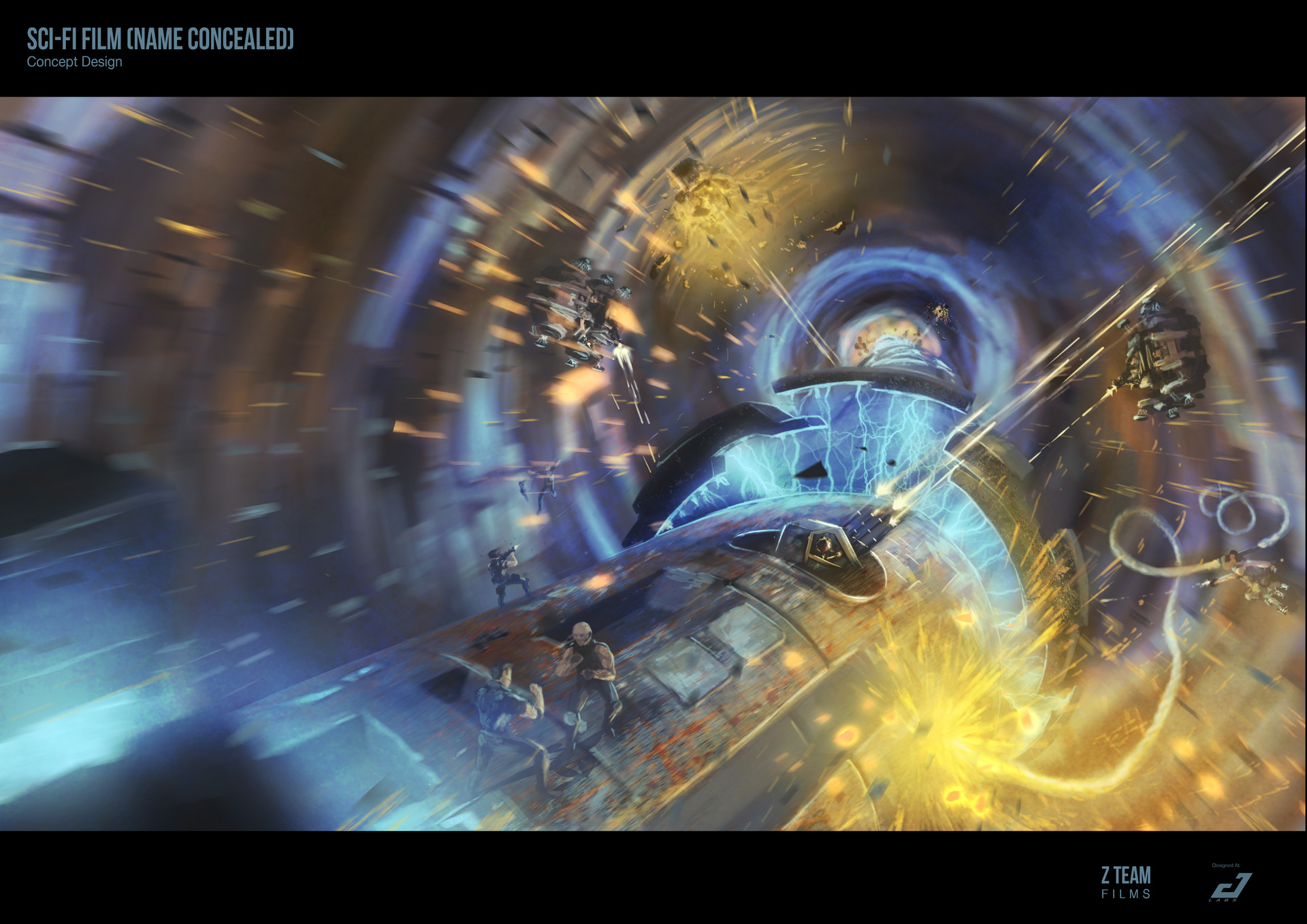The image is an electrifying and dynamic sci-fi concept art for a futuristic film. It depicts a chaotic scene of a spaceship hurtling through a wormhole or portal to another dimension, surrounded by vibrant blue lights and fiery orange and yellow explosions. The spaceship, heavily damaged by enemy fire, emits a flurry of bullets and ammunition towards two attacking ships. The setting resembles a swirling vortex or a virtual tunnel with circular walls, illuminated by various lasers and light streaks.

Amidst the intense battle, two men in combat stances are seen atop a massive silver cylinder or rod that serves as a floor. One man, bald and wearing a black shirt with blue jeans, faces off against another man with brown hair in a short-sleeved blue shirt and blue jeans. In the background, an individual in black army gear points a gun upwards, adding to the chaotic atmosphere of the scene dominated by light and sparks.

The image is framed by black borders, with the top left corner displaying the text "sci-fi film (name concealed)" and "concept design" beneath it. The bottom right corner features the logo and name "Z Team Films," along with a stylized emblem resembling the letter 'D' or 'J'. The background details are deliberately faded, ensuring the damaged spaceship and its intense surroundings remain the focal point of this vivid and action-packed illustration.